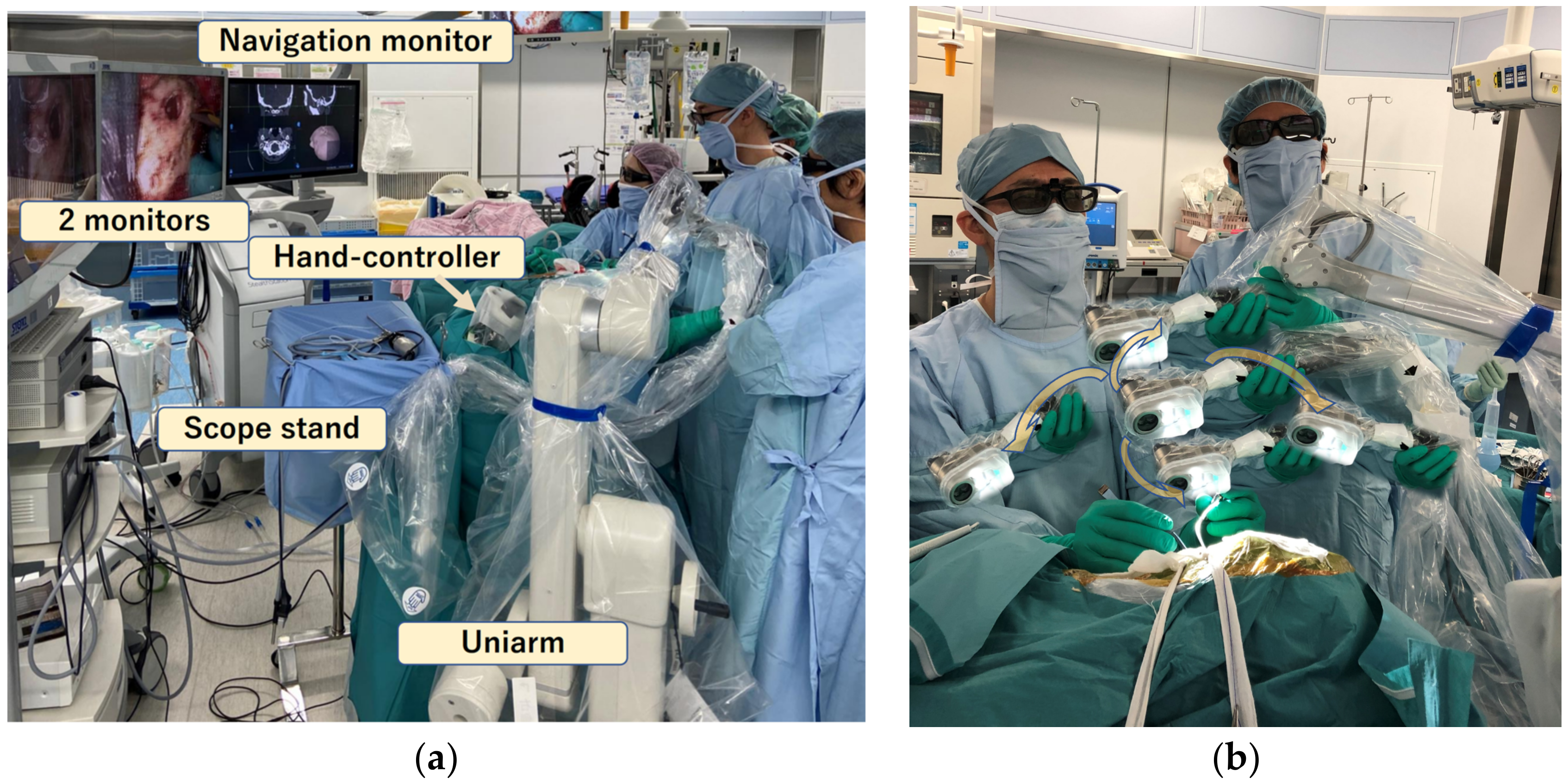Side-by-side images labeled A (left) and B (right) showcase a detailed view of a surgical suite during a robotic surgery. In Image A, the scene captures four fully gowned medical personnel in blue scrubs, masks, and surgical caps. They are immersed in a complex procedure, focusing on various pieces of high-tech equipment labeled for clarity. At the top, a "Navigation Monitor" is displayed, followed by "Two Monitors" beneath it, and a "Hand Controller" near the patient. Lower yet are labels for a "Scope Stand," and at the bottom right, an impressive "UNA Arm" wrapped in plastic. The room, clad primarily in gray and white, is bustling with activity as everyone pays close attention to the monitors reflecting the internal view of the patient.

Image B shifts perspective to a close-up of two surgeons, still in the same scrubs, but now clearer in detail with their green surgical gloves and additional eye protection, previously unnoticed sunglasses. This angle offers a more intimate look at the teamwork, including several extra hands out of frame, all operating around numerous pieces of camera equipment while the patient lies prone beneath them. The striking attention to detail and the sterile, high-tech environment underscore the precision and collaborative effort essential in modern surgical procedures.